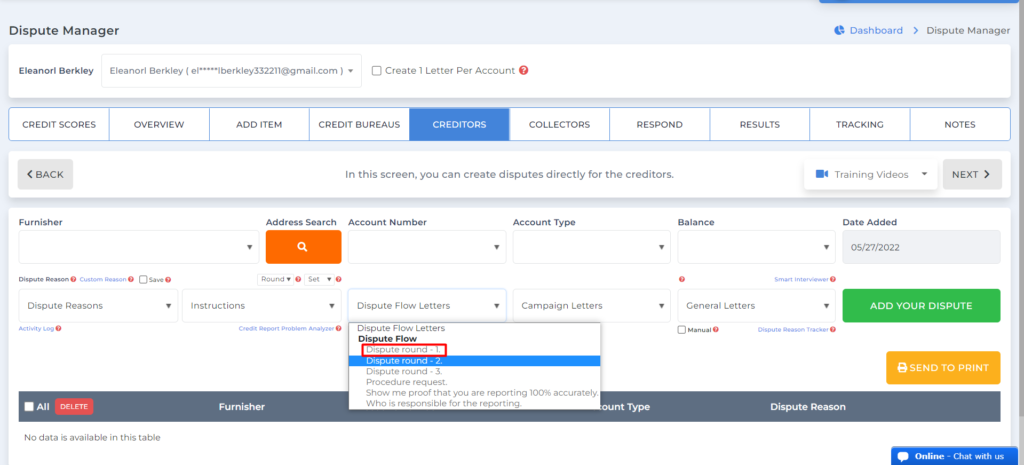Screenshot of the DisputeManager Software Interface

In this detailed screenshot of the DisputeManager software interface, the active page is prominently marked with the title "DisputeManager" in bold text within the header section. To the right of the title, a breadcrumb navigation trail indicates the user's path from the Dashboard to DisputeManager. 

Directly beneath the title, the interface displays user information, identifying the user as Eleanor Berkeley, with the email address eleanorberkeley332221@gmail.com. An option to create one letter per account is available via an unchecked checkbox.

The interface features several navigation tabs, including Credit Scores, Overview, Add Item, Credit Bureaus, Creditors, Collectors, Respond, Results, Tracking, and Notes. The "Creditors" tab is currently active, as indicated by both the highlighted state and the accompanying message below the tabs, which reads: "In this screen, you can create disputes directly for the creditors."

On the right side, buttons for accessing training videos and a "Next" button are immediately noticeable, offering additional support and navigation options. Below this section, the user can engage with the form search functionality.

The form search comprises input fields where users can enter details to create a dispute. This includes fields for furnishing information via a dropdown menu, address search, account number, account type, balance, and date added (notably displayed as 5/27/2022). Users can select a dispute reason from the provided options, guided by instructions showing the "Dispute Float Letters" dropdown menu, which presents options such as 1, 2, and 3 for selection.